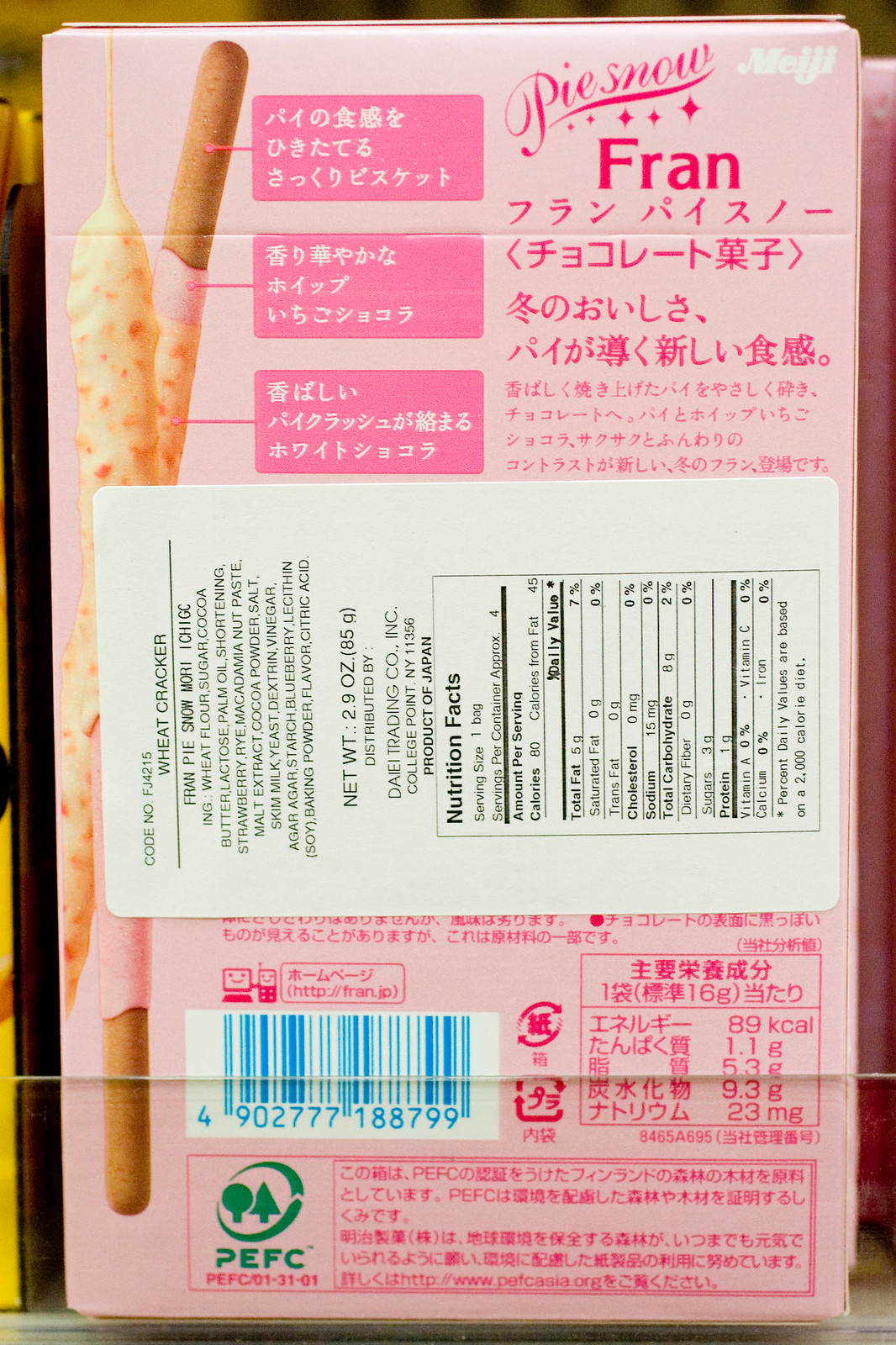This photograph features the backside of a cardboard food container, specifically designed for a type of long, skinny breadstick cracker. The container is predominantly light pink and adorned with dark pink text in Asian characters. To the left of the container, there's an image showcasing the actual breadstick cracker, which has been dipped in a pink-colored white chocolate coating, sprinkled with small crunchy bits. Centered on the box is a prominent white label with black text, which is placed sideways. This label contains both English text and a nutritional facts section. Additionally, there is a blue and white barcode positioned toward the bottom of the box, providing more product information.